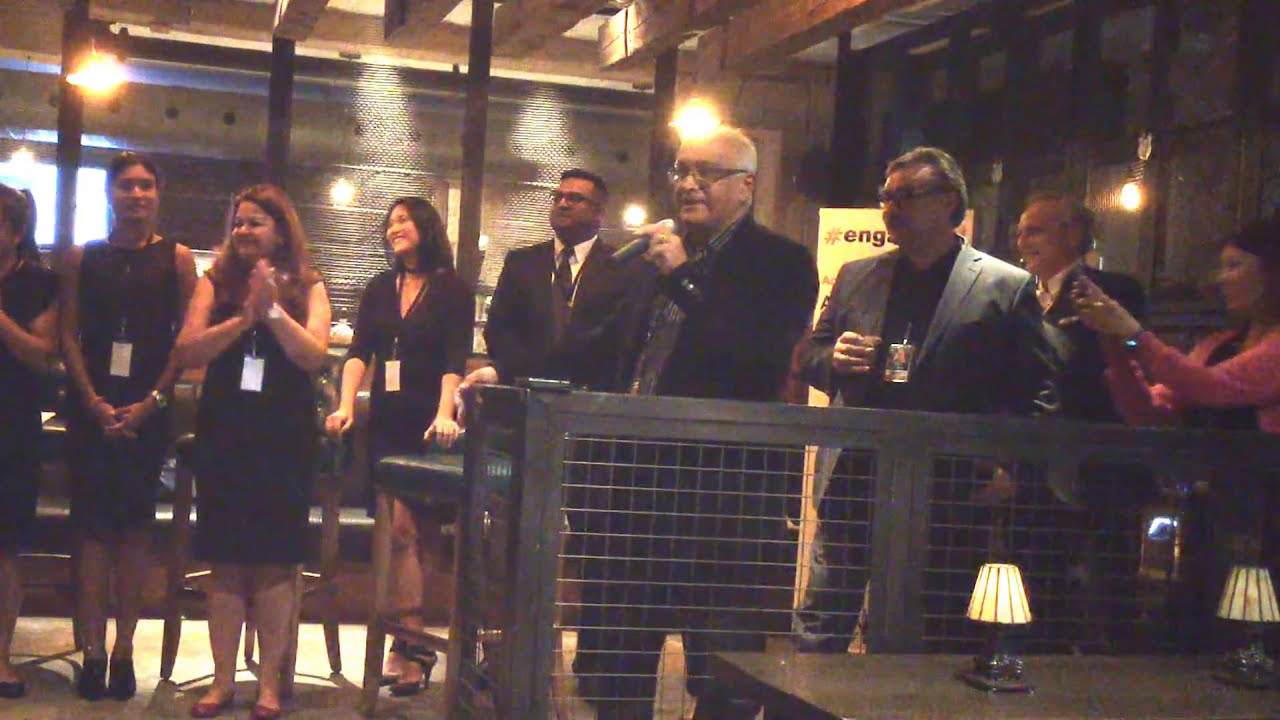This image captures a lively gathering of elegantly dressed individuals in what appears to be a modern, industrial-themed bar, possibly for an office party or a retirement celebration. The room is framed with wooden paneling and large windows adorned with dim lighting, creating a cozy yet sophisticated ambiance. Several people wear lanyards with IDs, indicating a formal or corporate event. 

In the foreground, an older man with gray hair and glasses, dressed in a business suit, holds a microphone in his left hand. He seems to be giving a speech or making an announcement, as indicated by the smiles and attention of the crowd. Behind him, another man in a gray suit coat holds a cocktail, adding to the festive atmosphere. Tables behind a stylish fence feature small cocktail lights, contributing to the modern design of the space, marked by glass, metal, and wood beams.

To the left, three women dressed in black party dresses and high heels stand with lanyards and IDs, engaged and smiling at the ongoing presentation. Among them, one woman is clapping, further suggesting a celebratory or award-giving context. On the right, more men in suits, some with ties, observe and enjoy the event. There's even a woman in pink capturing the moment with a camera, underscoring the significance of the occasion. The overall scene is one of joy and camaraderie, set against a backdrop of sleek, modern architecture.